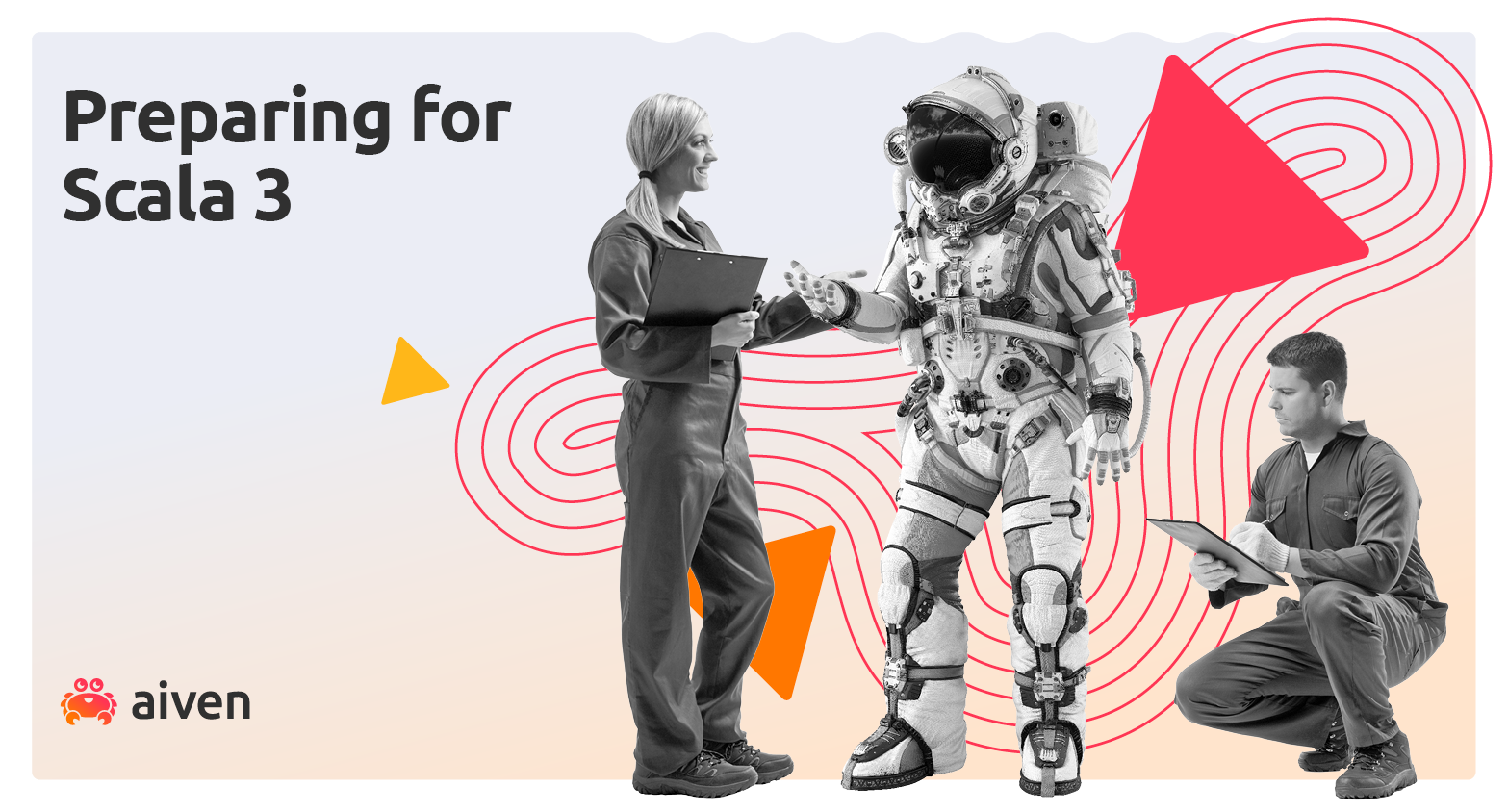This image is a detailed flyer for a tech company, AIVEN, promoting "Preparing for Scala 3." The flyer is rectangular in shape with a digital geometric background featuring an off-white base with swirling pink lines and geometric shapes in pink, orange, and yellow. The primary colors in the design include black, white, yellow, orange, red, pink, peach, and gray.

In the center, the image showcases three people, depicted in black and white. On the left, a woman with a ponytail, dressed in a jumpsuit, holds a notebook and appears to be holding hands with an individual in full astronaut gear, including a dark-visored helmet and padded articulated joints. To the right, a man, also in a jumpsuit, is kneeling and writing on a clipboard.

The text "Preparing for Scala 3" is prominently displayed in black letters in the top left corner. In the bottom left corner, beside a vibrant logo featuring a crab in shades of orange, pink, and red, is the name "AIVEN" in black letters.

The overall style of the flyer combines photographic elements with a digital, geometric design, creating a visually engaging and modern aesthetic.